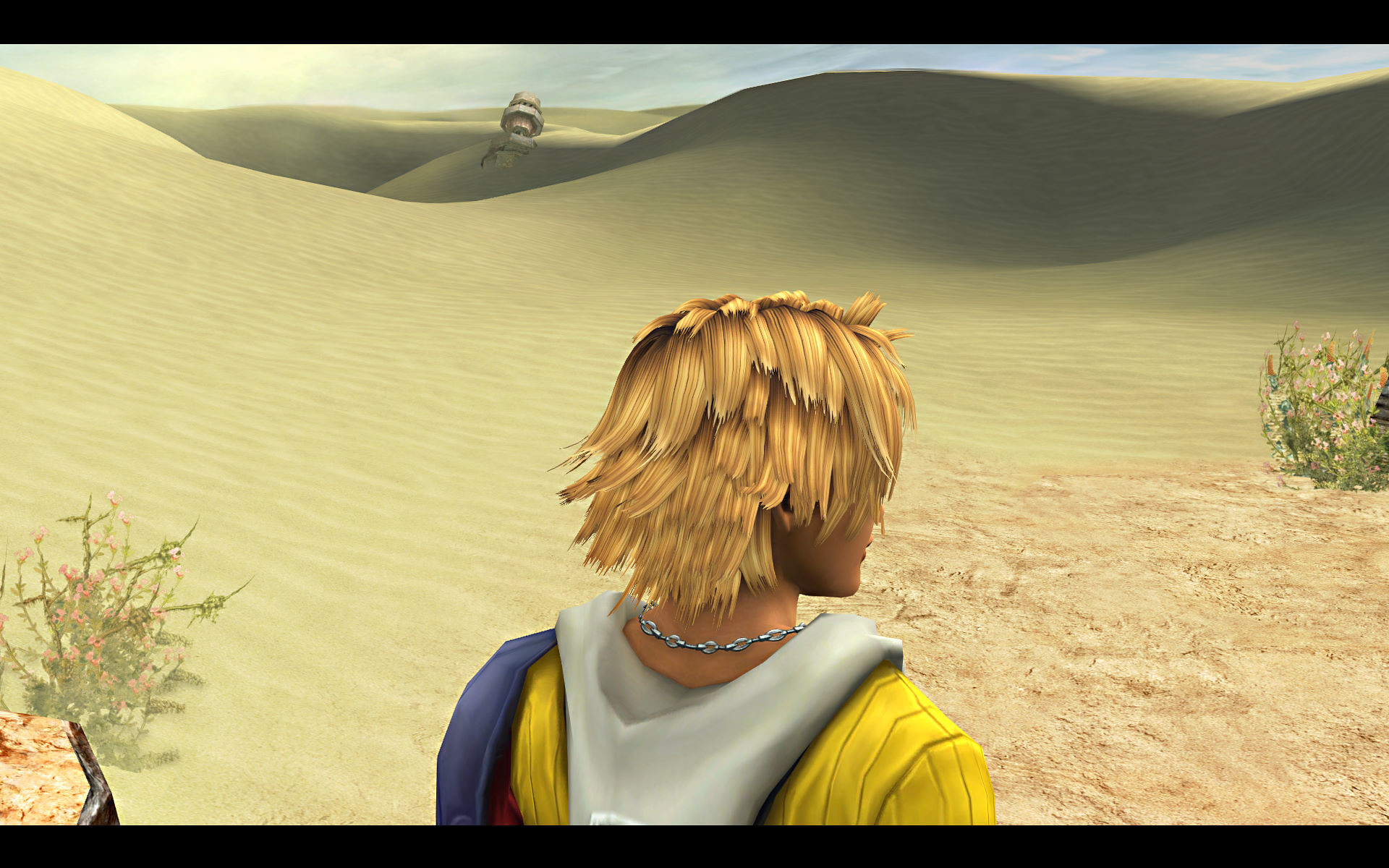In this digital artwork, we are presented with a captivating desert landscape characterized by light yellow sands and softly shaded dunes. The subtle gradient in the dunes, with darker tones nestled in the depressions, adds depth and realism to the scene. At the base center of the image, we see the back of a young individual, gender indistinct, donning a yellow shirt. Their jaggedly cut blonde hair reaches the nape of their neck, with long bangs partially visible. They stand gazing east, offering a glimpse of their profile – a chin, a touch of the nose, and the outline of their mouth are faintly discernible. The person also sports a silver chain choker necklace that catches the light subtly. In the lower left corner, there is a dry, weathered plant sprouting pink flowers, while a similar plant, also adorned with small pink blossoms, appears mid-section on the right side. This intricate digital artwork merges the serenity and harshness of the desert in a beautifully composed scene.